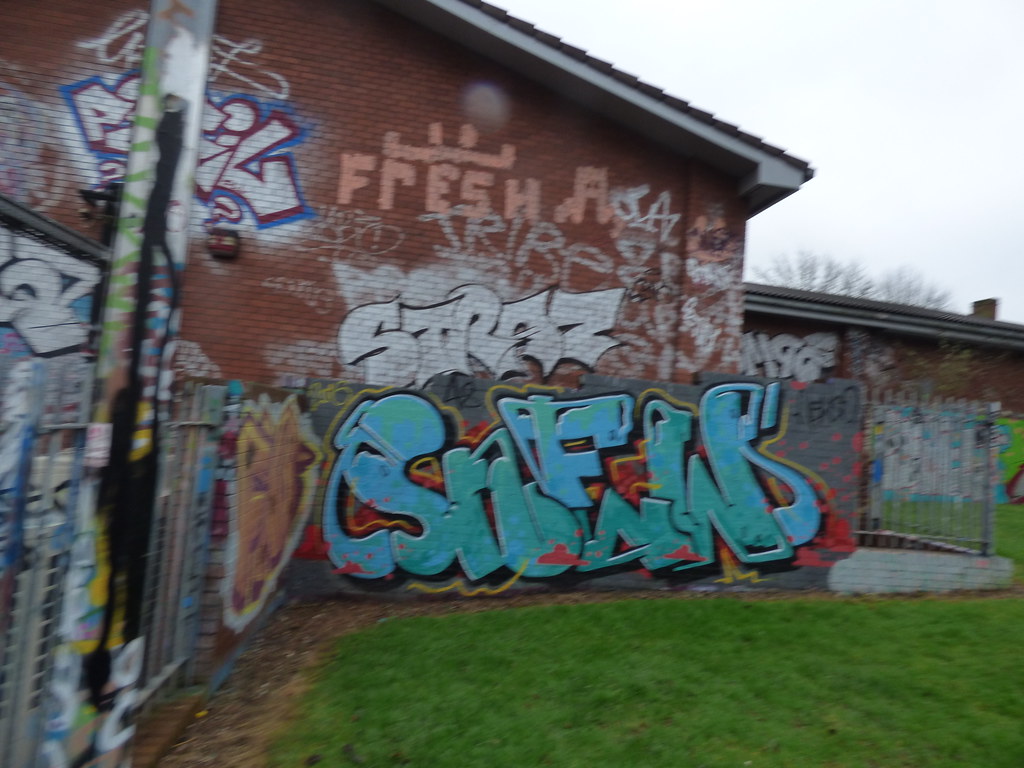In this slightly out-of-focus color landscape photograph, we see the side of a red brick building adorned with extensive and intricately crafted graffiti. The building's pitching roof extends upwards to the left, but its top is cut off due to the framing of the image. The red brick wall, as well as a separate wall in front of it, are entirely covered with diverse styles of graffiti, predominantly in bubble-style letters with vibrant colors ranging from blues to whites to flesh tones. Much of the graffiti includes various words and phrases, though some are partially illegible. Notably, there is a highly detailed mural that appears skillfully painted with clean lines and smooth color blending, suggesting a significant level of artistry.

To the left of the frame, metal railings extend at a 90-degree angle from the wall, both the railings and the metal lamppost in the foreground are also adorned with graffiti and show signs of wear and rust. Below the building, a small patch of lush green grass adds a touch of nature to the urban setting, accompanied by a brown area of earth or mulch in front of the wall.

In the back right, another red brick structure with a horizontal roof, similarly covered in graffiti, can be seen. Above this building, treetops encroach into the scene under a clear whitish light grey sky, indicating the photo was taken during daytime. The overall atmosphere suggests an overcast day, intensifying the urban ambience of graffitied architecture and metal structures contrasted by patches of greenery.